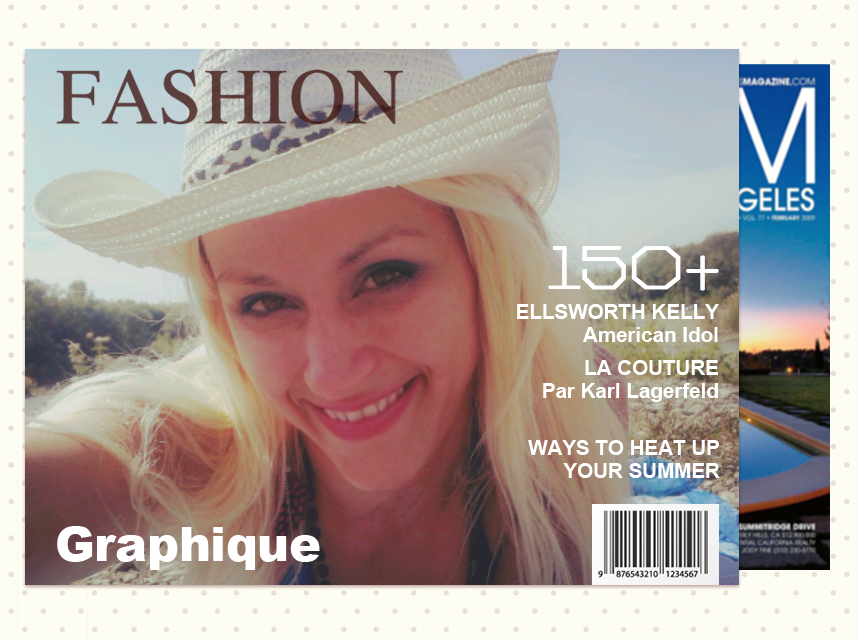The image features a vibrant fashion magazine cover set against a yellow background adorned with brown polka dots. Dominating the foreground is the magazine titled "FASHION," prominently displayed in bold, capitalized brown letters at the top. The cover headlines include "150+," "Ellsworth Kelly," "American Idol," "LA Couture," and "Karl Lagerfeld," alongside a feature titled "Ways to Heat Up Your Summer." A barcode is positioned in the lower right-hand corner, and "Graphique" is clearly printed on the lower left.

In the background, a blonde woman with bleached hair and expressive makeup—comprising pink lipstick, heavy eyeliner, mascara, and black eyeshadow—smiles at the camera, revealing her top teeth. She wears a striking white cowboy hat adorned with a leopard print design. Slightly visible in the background to the right edge of the main magazine is another magazine cover, though its details remain indistinct.